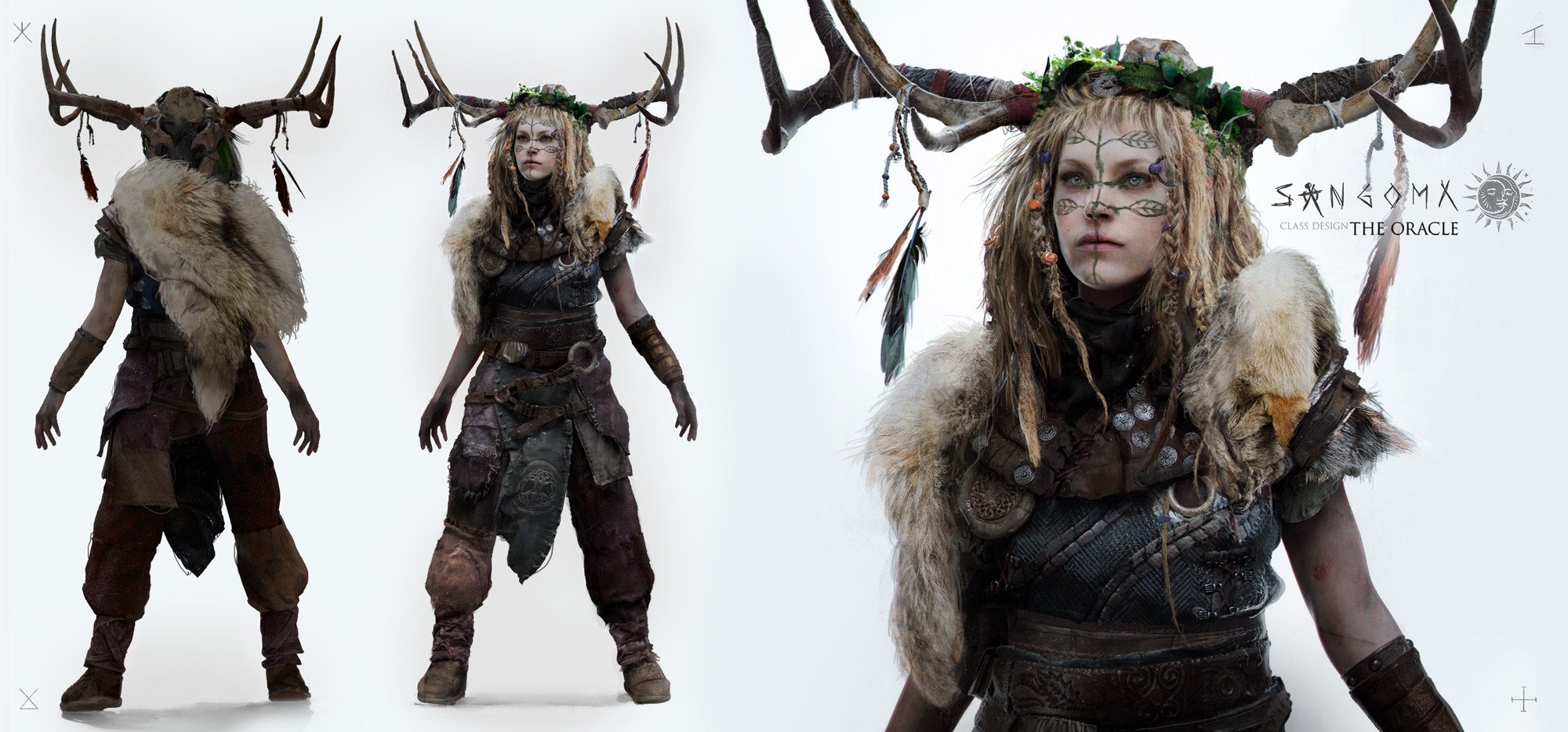The composite image features three views of a woman dressed in elaborate, ancient-inspired costume. The central and right images show her from the front, while the left image displays her from the back. She is adorned with an intricate headpiece made of large antlers embellished with flowers and dangling feathers. Her face is painted with leaf-like designs, possibly serving as camouflage. Her hair is styled into thick braids and dreads, interwoven with colorful beads. She wears a rugged, handmade-looking outfit consisting of animal pelts around her shoulders and a leather ensemble that includes a warm-looking jacket, belted pants, and large boots. Her left arm is wrapped in a leather bracer. The right image focuses on her upper body and face, showing more detail of her headpiece and facial decorations, while the central image provides a full-body view. The text in the upper right corner reads "Sango Mix. Class Design The Oracle."